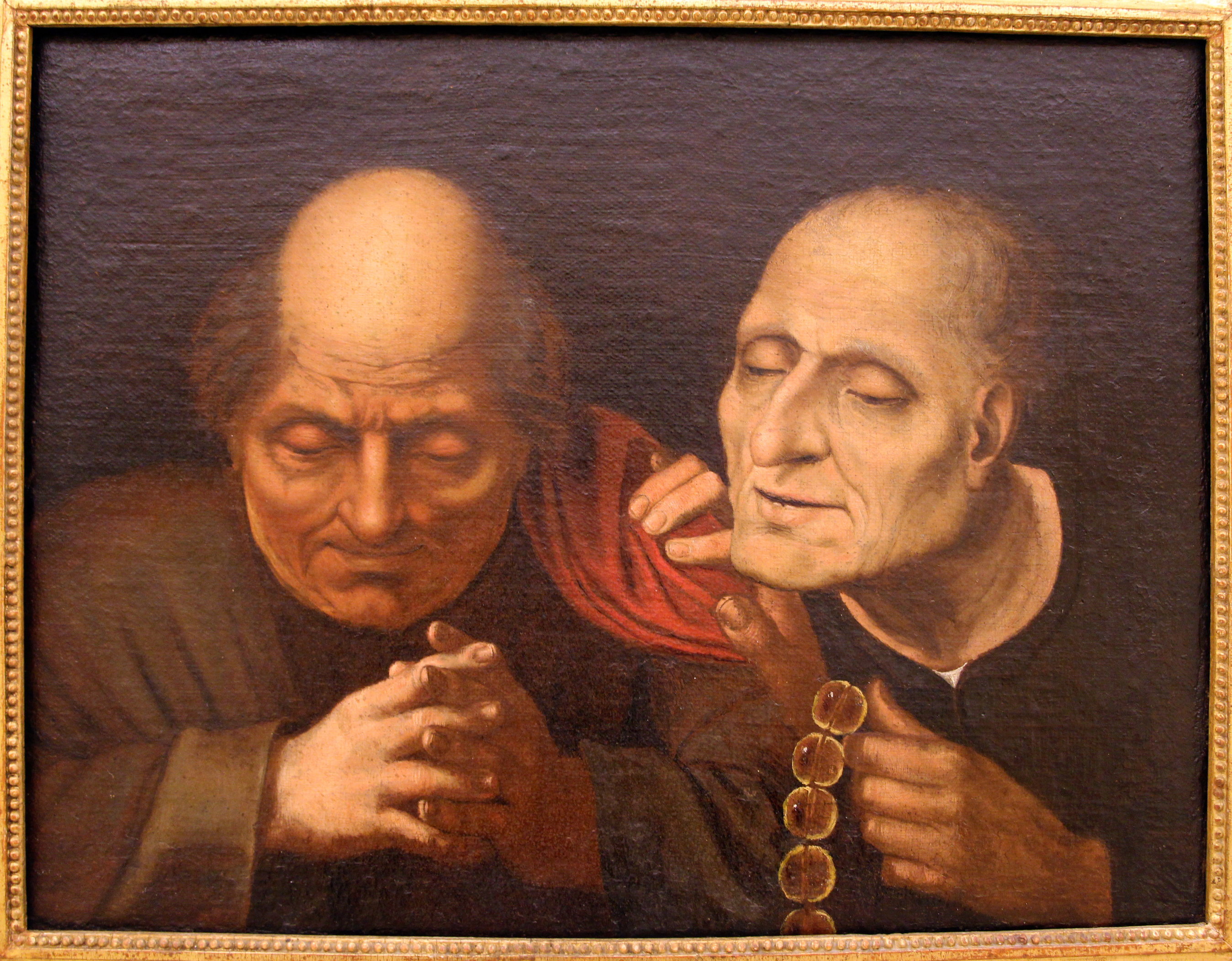This photograph captures a painting encased in a gold frame, presenting a tranquil scene set against a dark, almost black, background. The painting prominently features two elderly men engaged in a moment of contemplative prayer. The man on the right, dressed in a dark brown robe with a distinct white collar at the neckline, holds a rosary with brown beads in his left hand. His right hand rests gently on the left shoulder of the second man, who stands to his left. This second man, attired in a brown robe with a red cloak draped over his left shoulder, has his fingers intertwined and his head bowed slightly, his eyes partially closed in quiet reflection. The peaceful expressions and serene postures of both men, with the right man's face upturned and the left man's head bowed, convey a deep sense of devotion and calm. The painting is unsigned and undated.